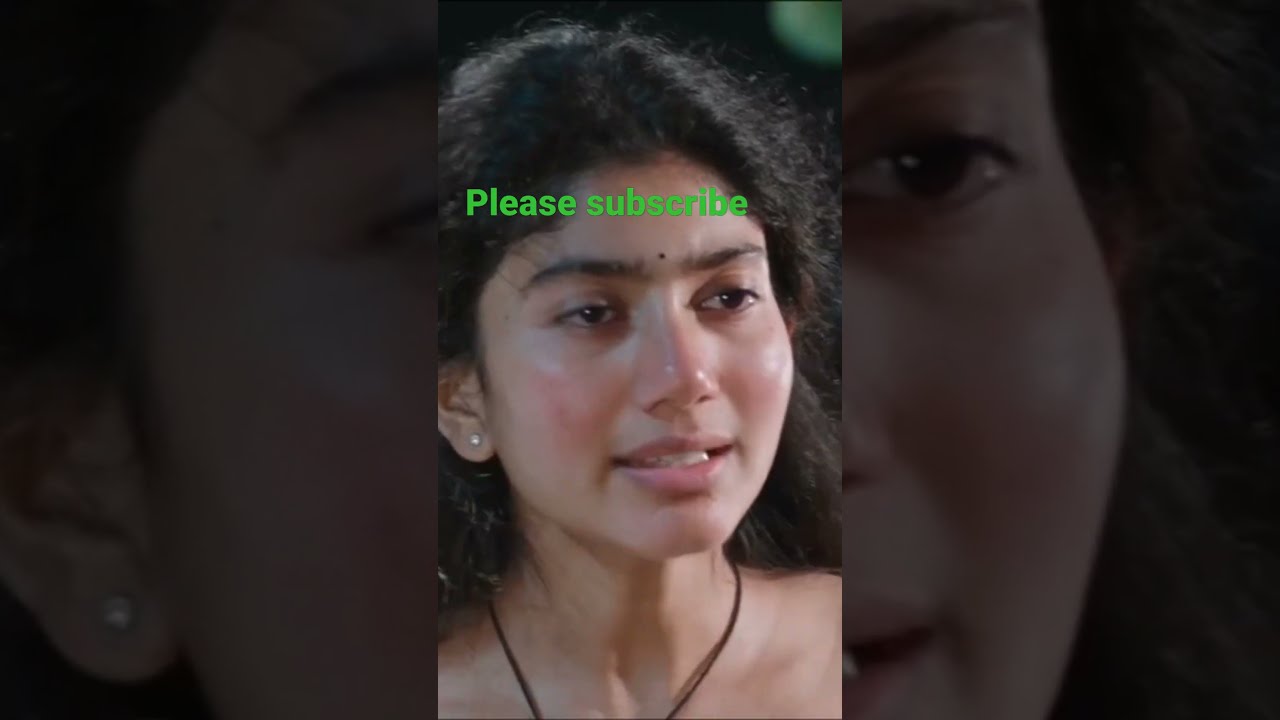The image features a closely framed, photorealistic portrait of a woman with an intriguing composite background. The central section of the image showcases the woman's face from the top of her shoulders to the top of her head. She has light brown skin, deep brown eyes, and striking dark, curly or wavy hair. Her pronounced dark eyebrows draw attention to her expressive eyes, which gaze towards the right. A small black dot sits prominently between her eyebrows. She wears bright white or possibly diamond earrings and a minimalist black string necklace. Her expression is subtle, with her mouth slightly open, revealing a hint of her teeth in a soft, almost half smile.

The central portrait is flanked by the same woman's zoomed-in and darkened visage in the background, creating a layered effect that adds depth to the composition. This background is less transparent than the central image, emphasizing the primary focus on the woman. The background image blurs the details but maintains the outline of her face and hair, giving a cohesive but mysterious touch to the overall scene. Over her forehead in the central image, bright green block text boldly states, "please subscribe," adding a modern, interactive element to the visual narrative.